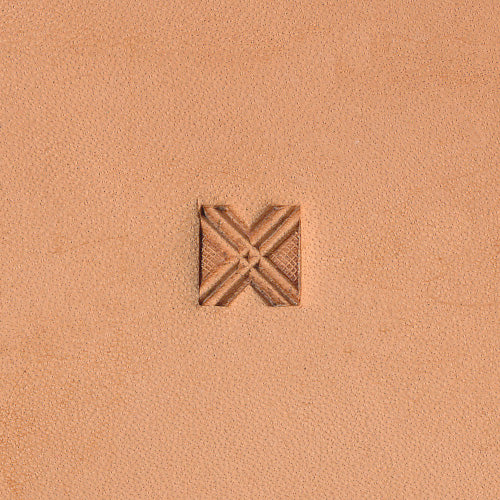The image depicts a close-up view of a makeup palette featuring a soft, light tan surface with a uniform texture. At the center, there is a distinctive, square-shaped indentation resembling a small, brown X. This X pattern consists of two intersecting lines at 45-degree angles, creating a subtle honeycomb pattern within the left and right sections. The surrounding palette surface is consistent in color and texture, suggesting a makeup product such as eyeshadow or blush. The detail and precision of the central X pattern give the impression that it might have been purposefully stamped or designed into the material.